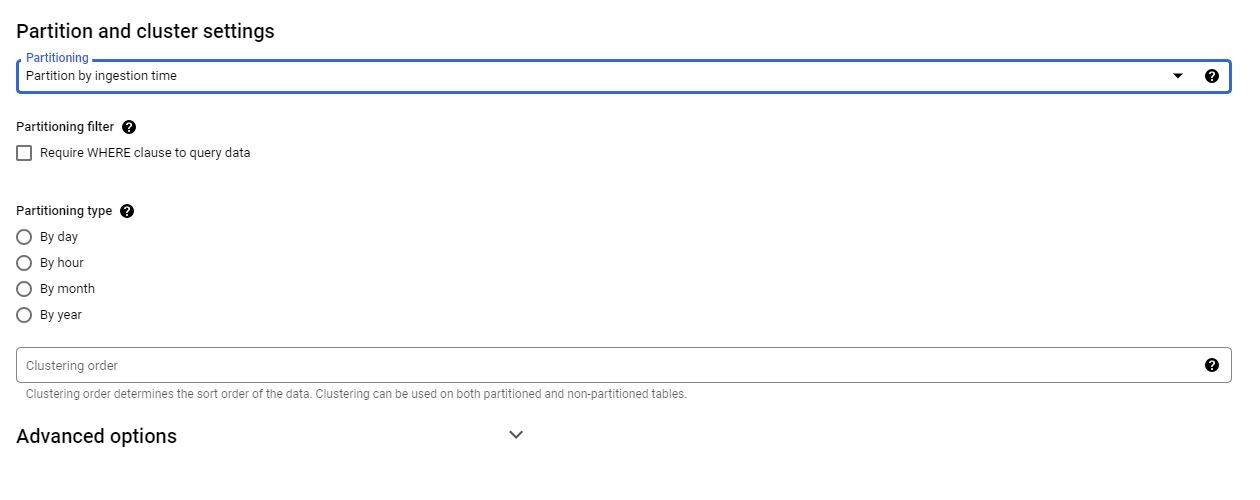The horizontal rectangular image features a user interface for configuring partition and cluster settings. At the top, the title "Partition and Cluster Settings" is displayed in a small, bold, black font, with only the word "Partition" capitalized. Beneath the title, a prominent horizontal rectangular box outlined in dark blue spans the width of the image. Within this box, at the left edge, the word "Partitioning" is printed in blue font. Inside the box, the text "Partition by Ingestion Time" is displayed in black font. 

On the right side of the box, there's a pull-down menu accompanied by a dark circle with a white question mark inside. Below this box, the text "Partitioning Filter" is written in black font, again with a question mark in a dark circle next to it. Directly under this, there's an empty square labeled "Require WHERE clause to query data," with "WHERE" fully capitalized.

Further down, the text "Partitioning Type," paired with another question mark in a dark circle, introduces a series of options for partitioning types. These options—"By Day," "By Hour," "By Month," and "By Year"—are each preceded by empty circles, indicating selectable options.

Another horizontal rectangular box stretches across the image, containing the faint text "Clustering Order." To the right of this text is yet another question mark. Under this, descriptive text reads, "Clustering order determines the sort order of the data. Clustering can be used on both partitioned and non-partitioned tables." Finally, a downward arrow appears beneath this description, and in bold font on the left, the phrase "Advanced Options" is displayed.